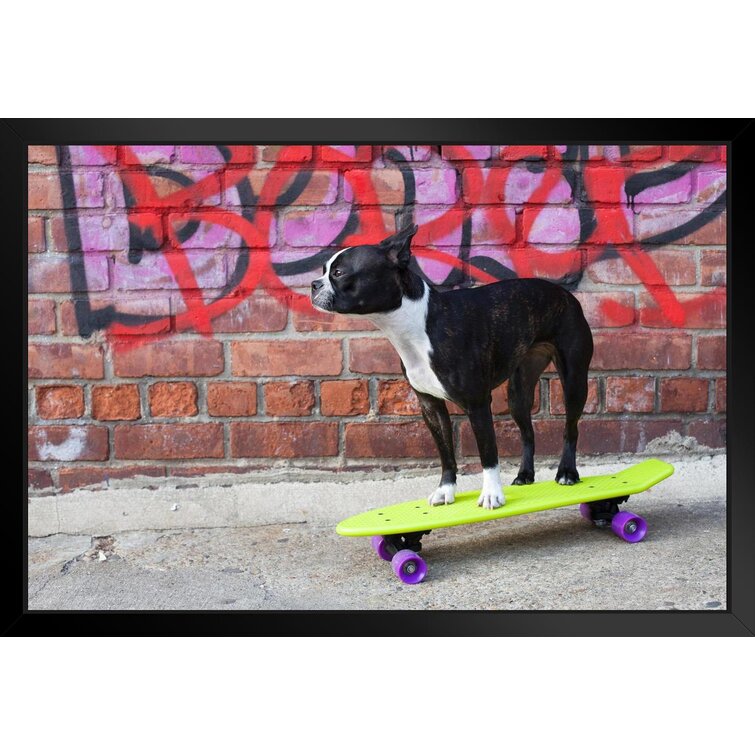This photograph features a small black dog with a white chest, white front paws, and white markings under its chin and between its nose. The dog is standing, appearing relaxed and chilled out, on a neon green skateboard with purple wheels. The skateboard is stationary on a cement floor set against a classic red brick wall in what appears to be an urban alley. The wall is adorned with intricate graffiti, including a prominent purple tag with a black outline, partially overlaid with red graffiti. A small black border frames the photograph, adding a polished touch to the overall composition.